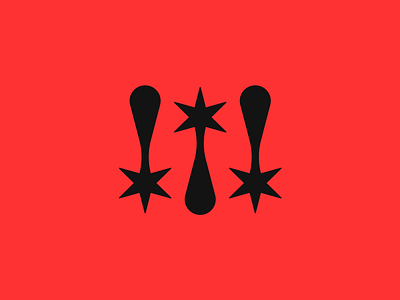The image portrays a minimalist graphic design with a bright, primary red background. Centrally positioned are three black silhouettes. The middle silhouette features a five-pointed star at the top, with a vase-like base beneath the star, resembling a utensil handle or the elongated form of a conical structure that ends in a rounded base similar to a baseball bat’s head. Flanking this central figure, the silhouettes on both the left and right are identical to the central one but are flipped upside down. These symbols are purely black with no additional details, creating a stark contrast against the red backdrop. The entire design maintains symmetry, with equal sizing for all three elements, suggesting a flag-like simplicity and geometric precision.